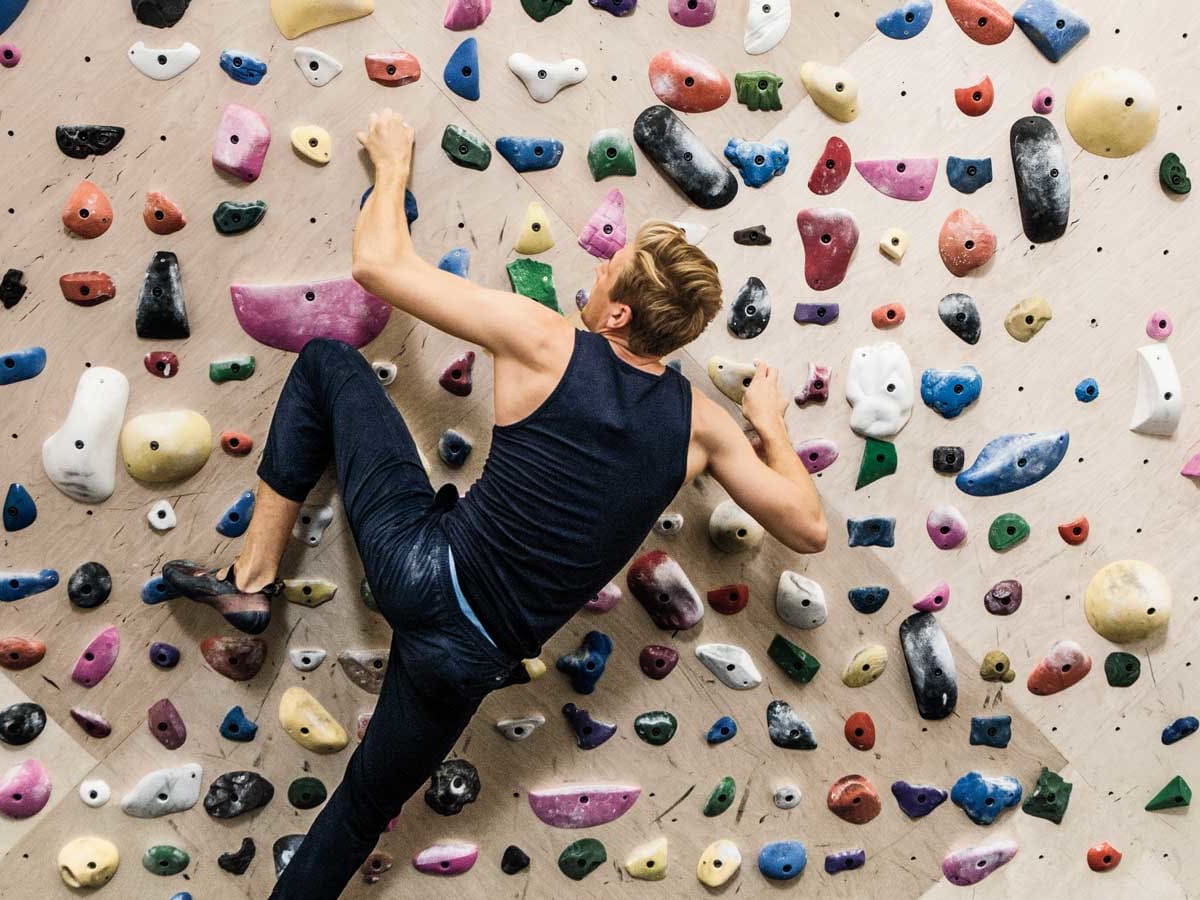In this professionally captured indoor photograph, we see a man climbing a meticulously designed rock climbing wall made of wood. The wall is densely adorned with an array of brightly colored holds, including shades of dark green, dark blue, light blue, orange, red, black, white, green, and purple. These holds, varying in shapes and sizes from 1 inch to 10 inches, create an intricate pattern reminiscent of jewels embedded in the wall. The climber, a light-skinned individual with brown hair, is equipped with black climbing shoes, which seem to lack prominent soles, hinting at a specialized design, along with black and tan leather booties. He wears dark blue pants and a black sleeveless tank top, showcasing his physically fit form. The man is positioned about 80% up the wall; his left hand is reaching three rows from the top, while his right hand is about six rows down. His feet and hands are securely planted on various holds, amid the vivid texture and detail of the climbing surface. The image is shot with exceptional clarity and lighting, emphasizing the tactile quality of the wall and the intense focus of the climber.